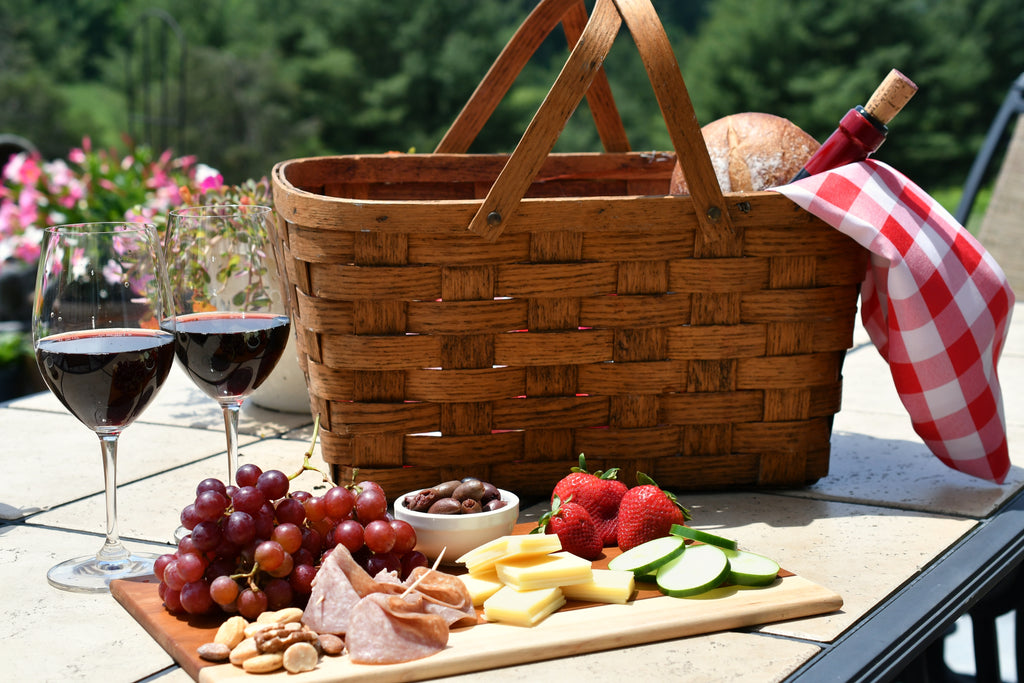In the photo, we are presented with a detailed close-up scene of a picturesque outdoor picnic set on a black and brown tiled table. The setting is vivid with the greenery of trees, patches of green grass, and a few pink flowers visible in the background, creating a serene and inviting atmosphere. 

At the center of the image is a large, woven wicker picnic basket with sturdy wooden handles. The basket is adorned with a red and white checkered cloth peeking out, evoking a classic picnic vibe. On the right side of the basket, the top of a wine bottle is visible, adorned with a purple burgundy foil, with its cork partially pulled out. Adjacent to the basket, we see the top half of an untouched, crusty, round loaf of bread.

To the left of the basket, two long-stemmed wine glasses are positioned side by side, each half-filled with dark purple wine. The glasses elegantly narrow at both the bottom and top, enhancing their refined appearance.

In front of the picnic basket, a small cutting board serves as a charcuterie platter, elaborately arranged with a variety of treats. Among these are bunches of purple grapes, a selection of yellow cheeses, slices of cucumber or zucchini, fresh strawberries, and an assortment of nuts. Additionally, a tiny white bowl holds Kalamata olives, contributing to the array of textures and flavors present on the board.

The bright, sunny ambiance adds a charming and warm touch to the well-prepared picnic tableau, making it a feast for both the eyes and the palate.